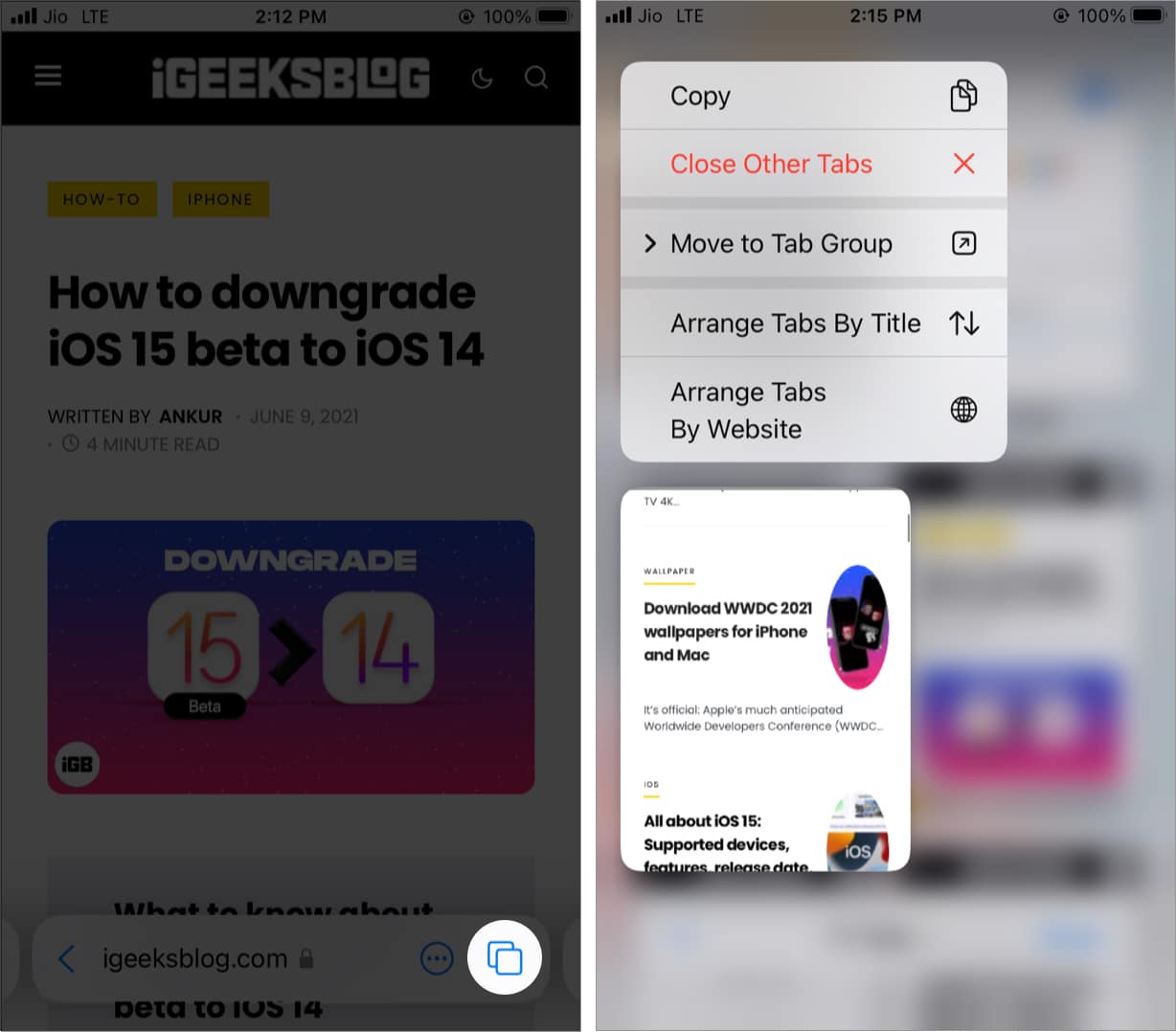The image presents two side-by-side screen captures from a digital platform, likely a smartphone or tablet interface. 

On the left side, there is a slightly dimmed screenshot of a website called "iGeeksBlog". The webpage prominently features an article titled "How to Downgrade iOS 15 Beta to iOS 14."

On the right side, another screenshot displays a series of pop-up menu options, including "Copy," "Close," "Other Tabs," "Move to Tab Group," "Arrange Tabs by Title," and "Arrange Tabs by Website." Below this menu, a smaller pop-up window lists two articles: "Download WWDC 2021 Wallpapers for iPhone and Mac" and "iOS 15 Supported Devices: Features, Release Date."